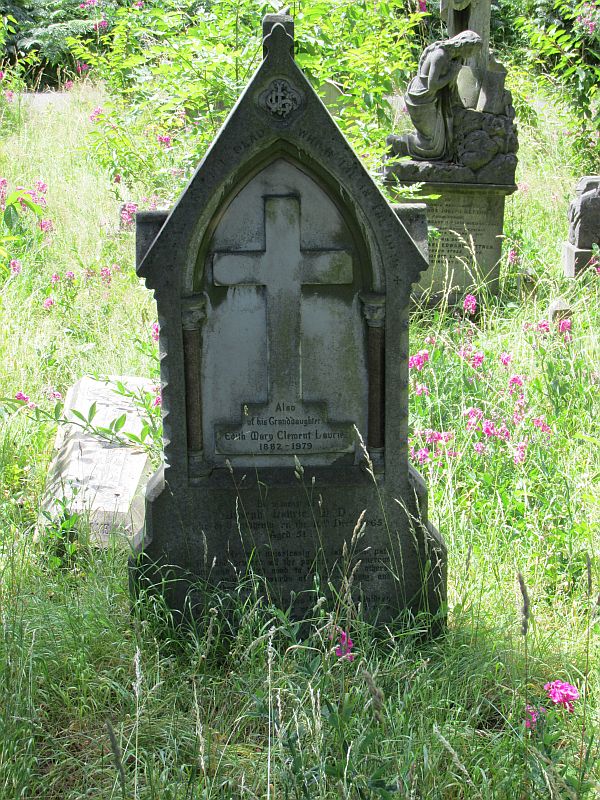This high-resolution photograph captures an overgrown cemetery characterized by tall green grass interspersed with vibrant pink and purple wildflowers. Dominating the foreground is an upright, weathered dark gray tombstone from 1882 that has been worn down by the elements. Its design is notable for its triangular top, reminiscent of a house with a roof and a rectangular body. The tombstone features an illegible inscription possibly starting with "Alex" or "Leo," and prominently displays a cross, which stands out in a lighter gray shade. Further back in the image, there are additional aging tombstones, including one adorned with a statue of a robed woman kneeling in prayer. The entire scene evokes a sense of history and serenity, underscored by the untamed vegetation that has reclaimed the cemetery grounds.